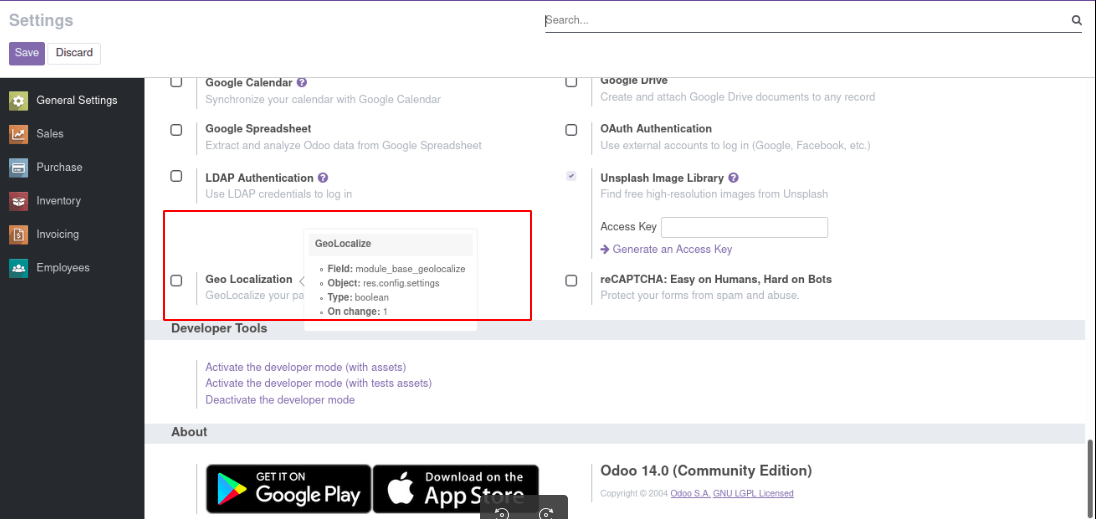The image depicts a user interface screen with a horizontal rectangular layout bordered by a light gray frame. Dominating the left side is a wide vertical navy blue banner, starting from the top with white text that reads "General Settings," and listing sequential options: "Sales," "Purchase," "Inventory," "Invoicing," and "Employees."

In the upper left corner of the screen, the heading "Settings" appears in light gray text. Beneath this heading are two distinct buttons: a purple button labeled "Save" in white letters, and a white button with purple text labeled "Discard."

The remaining right side of the screen features a white background divided into two columns at the top. The left column begins with the category "Google Calendar" in purple text, accompanied by a gray subtitle that reads "Synchronize your Calendar with Google Calendar." Below it is the "Google Spreadsheet" category, highlighted in purple with a gray subtitle stating "Extract and Analyze ODOO data from Google Spreadsheet," where "ODOO" is spelled out in uppercase letters. The final category in this column is "LDAP Authentication," in purple text with the description "Use LDAP Credentials to Login" in gray underneath.

The right column starts with the "Google Drive" category, followed by "OAuth Authentication," and "Unsplash Image Library," each in purple text. Below the "Unsplash Image Library" category, there is a text box designated for entering an access key.